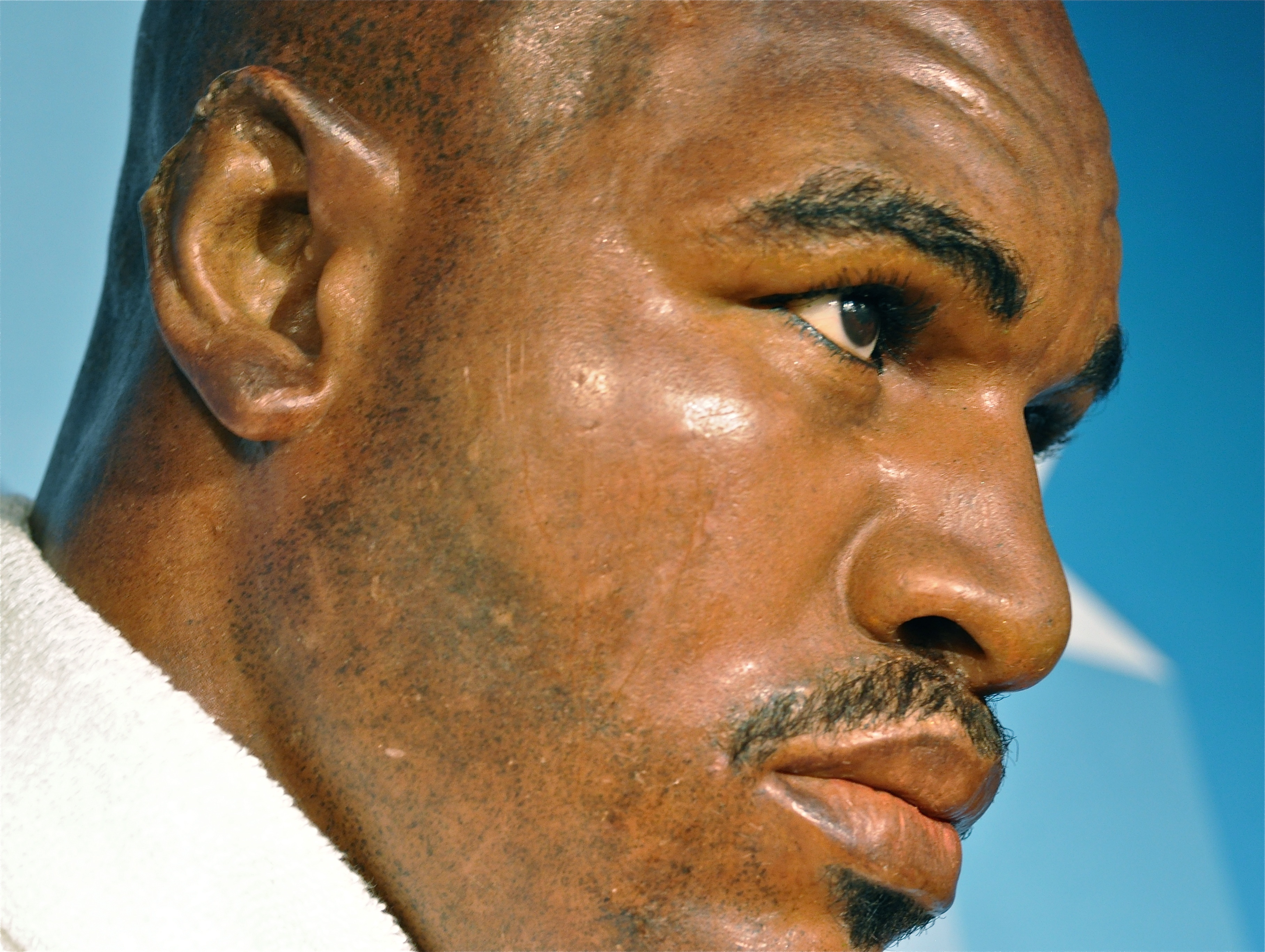This close-up photograph features Evander Holyfield, the renowned boxer, taken indoors against a blue and white backdrop that suggests a billboard or logo. The image focuses on the right side of his face, highlighting his distinct facial features. Holyfield, a black man, has a shaved head and sports a black mustache along with a small triangular goatee beneath his bottom lip. He is adorned with a white fuzzy material around his neck, likely the collar of a robe. His eyes are pointed upwards to the right, and he has a notably wrinkled forehead. A striking detail in the photograph is his right ear, which appears misshapen, with the upper part missing—an injury famously inflicted by Mike Tyson. The close-up captures his facial expression and the notable details of his right ear, emphasizing both his identity and his historic boxing injury.